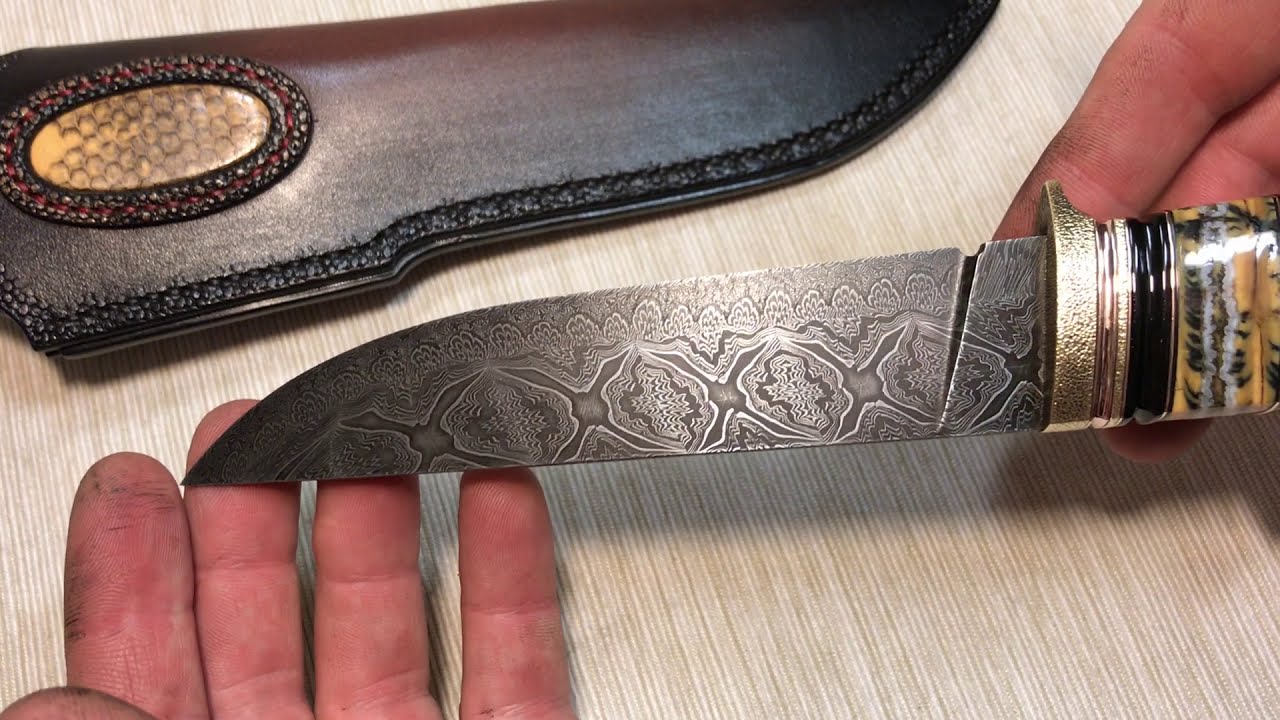This close-up image captures a highly ornate knife held by a person's hands, shown against a beige striped tablecloth background. The knife features a detailed Damascus-style blade with intricate silvery designs, including connected and half-circle patterns, giving it a matte yet glossy appearance. The handle is equally elaborate, adorned with a shiny pattern in yellow, green, black, and white hues, complemented by a brass gold hilt. The knife is held using two fingers on the right side at the base and four additional fingers laying flat on the left side, with the tip resting on them. Above, a leather sheath is visible in the top left corner, decorated with a prominent oval centerpiece. This ornate oval includes an amber-like jewel set into a honeycomb black pattern and is framed by a red-trimmed, raised ornate edge.